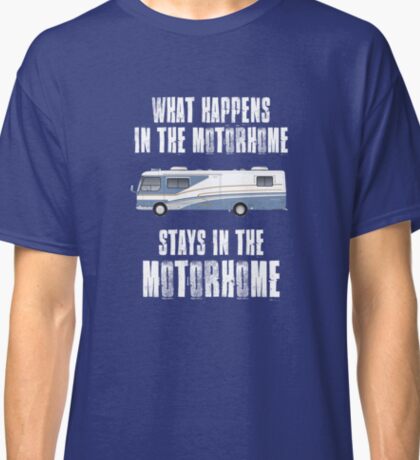This image features the torso of a man wearing a navy blue, short-sleeve, crewneck t-shirt. The t-shirt prominently displays a bold, eye-catching design across its center. In uppercase, off-white letters, it reads, "WHAT HAPPENS IN THE MOTORHOME STAYS IN THE MOTORHOME." An illustration of a long motorhome is seamlessly integrated into the text. The motorhome, colored white with blue stripes and some brown details, features distinct windows including the driver's seat window, a window just behind that, and a back window. The model's neck and arms are visible, suggesting a casual setting possibly intended for showcasing the t-shirt for sale, such as on a retail website. The overall composition is focused on clearly displaying the design on the t-shirt against the man's olive-toned skin.